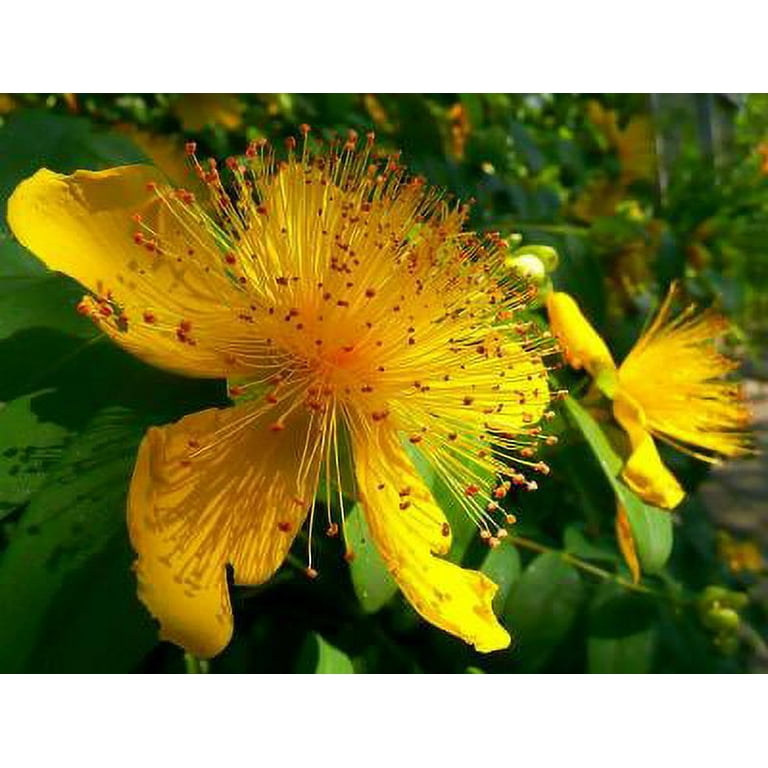This close-up photograph captures two prominent yellow flowers set against a blurred, green-dominated background, suggesting a natural, outdoor setting likely in a field. The foreground is primarily focused on one large yellow flower, slightly to the left of center, with a second similar flower slightly behind and to the right. The flowers, appearing to grow from a plant with large green leaves, display five to six crumpled petals that exhibit vibrant yellow hues with hints of orange. At the heart of the primary flower, numerous long yellow strands, each tipped with a red dot, extend outward. The image quality is relatively low-resolution, appearing pixelated due to significant zoom, and the strong sunlight creates noticeable shadows on the petals and leaves.